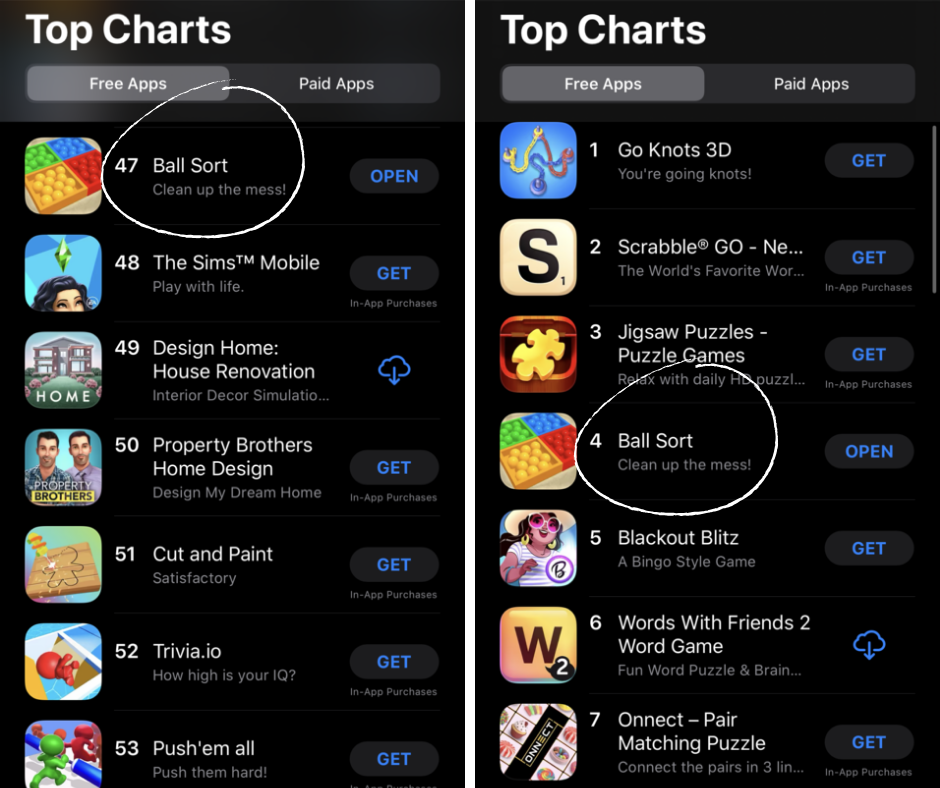The image features a black background showcasing a Top Chart list of apps, with the "Free Apps" section highlighted. The left side of the screen displays a list of games ranked from number 47 to 53:

- **47**: Ballsort (circled in red), with the tagline "Clean up the mess" and an "Open" button.
- **48**: The Sims Mobile.
- **49**: Design Home, House Renovation.
- **50**: Property Brothers Home Design.
- **51**: Cut and Paint.
- **52**: Trivia.io.
- **53**: Push Em All.

On the right side, still under the "Free Apps" category, the list continues, but with the higher-ranked apps:

- **1**: Go Knots 3D.
- **2**: Scrabble Go.
- **3**: Jigsaw Puzzles.
- **4**: Ballsort (circled again, previously listed as number 47 on the left).
- **5**: Blackout Blitz.
- **6**: Words with Friends 2, described as a board game.
- **7**: Onyx Pair Matching Puzzle.

The identical circled "Ballsort" appearing on both sides of the list highlights its intriguing placement disparity.